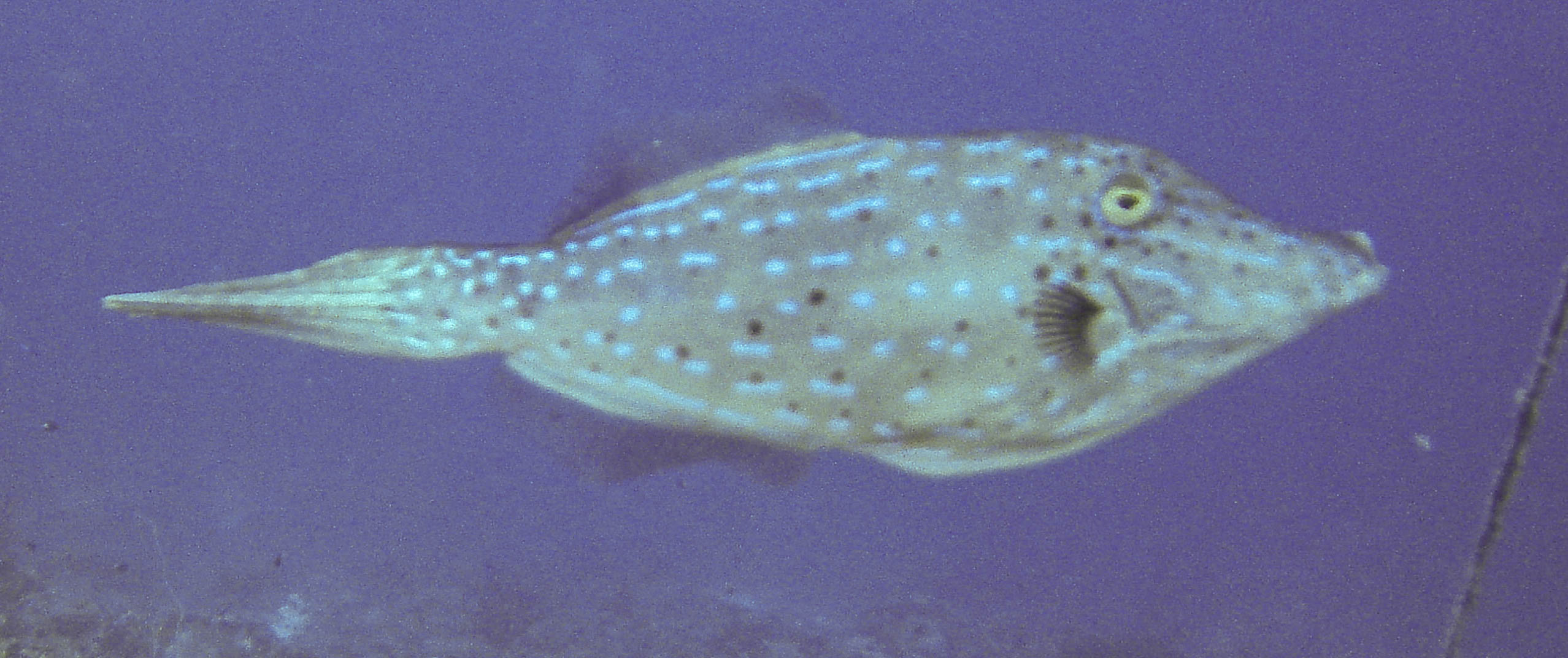This image features a fish swimming in a blue water background, which could be either a fish tank or the ocean. Centered horizontally in the picture, the fish head faces the right side. It has distinctive features including a pointy nose and a long, tapering tail that expands into a rectangle before narrowing again. The fish's body is adorned with irregular blue stripes and dash-like patterns along with black spots. Its eye is a striking yellow with a black pupil. The fish has several fins, including a prominent one on the top and another smaller one aligned near the bottom-left of its eye. Towards the bottom area of the image, there's some coral or ocean debris and a stick-like object extending from the bottom to the middle right. The underwater scene is characterized by a murky blue background.